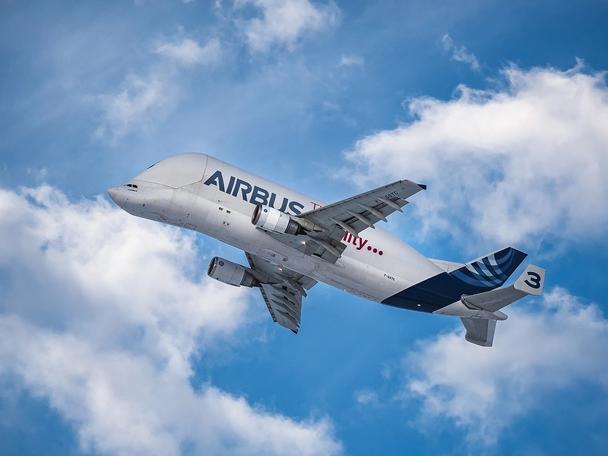The photograph showcases an unusual, white Airbus aircraft soaring in a vivid, saturated blue sky filled with fluffy white clouds. The plane, which appears smaller than typical commercial jets, exhibits a distinctive design with a very pointed and somewhat rounded nose cone. Two jet engines are situated beneath the midsection of its wings. The fuselage features partial lettering; prominently seen is the word "Airbus" in dark blue, while an obscured word ending in "ITY..." is visible in dark red. The rear of the aircraft is adorned with a large dark blue stripe, complemented by swirling white and light blue decorative elements on the tail. Notably, the tail’s fin bears the number 3 in navy blue. The absence of windows suggests it is not a standard commercial airliner, possibly modified for specialized transport, such as carrying a space shuttle.